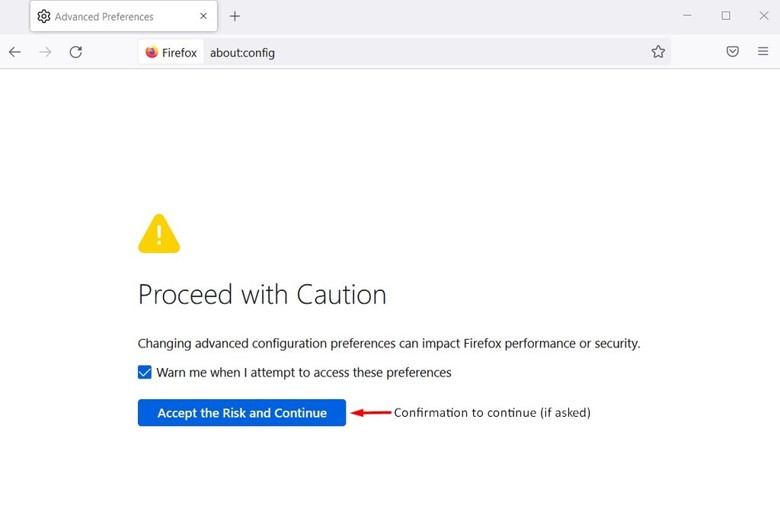A detailed screenshot of a Firefox configuration warning screen. The URL bar displays "about:config". Dominating the white background of the screen is a conspicuous yellow triangle with an exclamation mark, indicating a warning, positioned towards the left margin. Beneath this icon is a warning message in prominent dark blue text reading, “Proceed with Caution.” 

In standard-sized text below, a cautionary note states: "Changing advanced configuration preferences can impact Firefox performance or security." Adjacent to this text is a checkbox, already ticked, labeled: "Warn me when I attempt to access these preferences." 

Towards the lower section of the screen, there is a medium blue clickable button with white text that says, "Accept the Risk and Continue." Just to the right of this button, additional text in dark blue or bluish-gray reads: "Confirmation to continue, if asked." A red arrow points from the "Confirmation to continue" text towards the "Accept the Risk and Continue" button, emphasizing the action to be taken.